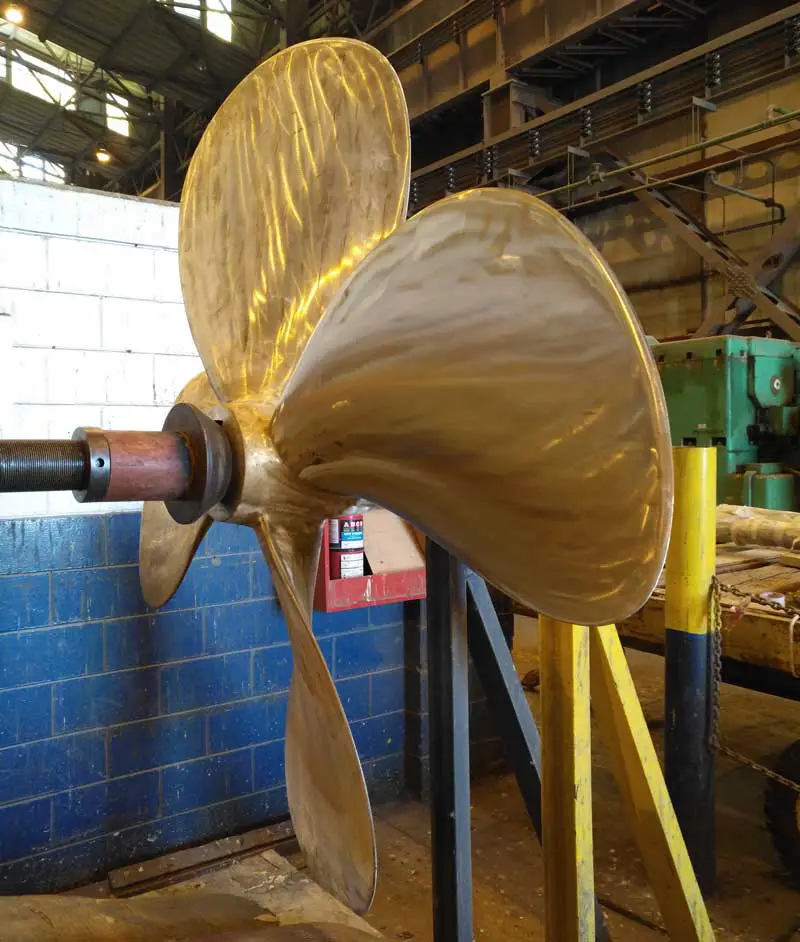In this image, we observe a large, four-bladed propeller with a distinct appearance. The propeller, mounted on a shaft extending to the left and off-screen, is primarily brown with noticeable streaks of yellow, suggesting a haphazard paint job over an originally yellow surface. The scene is set in what appears to be a warehouse environment, characterized by its unfinished concrete flooring and a partially deteriorated cement wall composed of white and blue bricks behind the propeller. The propeller is centrally positioned in the image, emphasizing its prominence and large size, which spans almost the entire height of the wall behind it.

Further details reveal a surrounding space filled with various industrial elements, contributing to the warehouse atmosphere. Visible are metal rails on the upper floors, metal stairs, and green machinery, along with a metal dumpster structure tucked behind the propeller. To the right of the propeller, caution poles with yellow tops and black bottoms stand out, presumably to prevent vehicular collisions within the warehouse. The setting is indoors, seemingly in the middle of the day, evidenced by the natural light illuminating the scene through high-set windows. The overall environment hints at a somewhat neglected state, with debris scattered and an old, worn look to the furnishings and structural elements.